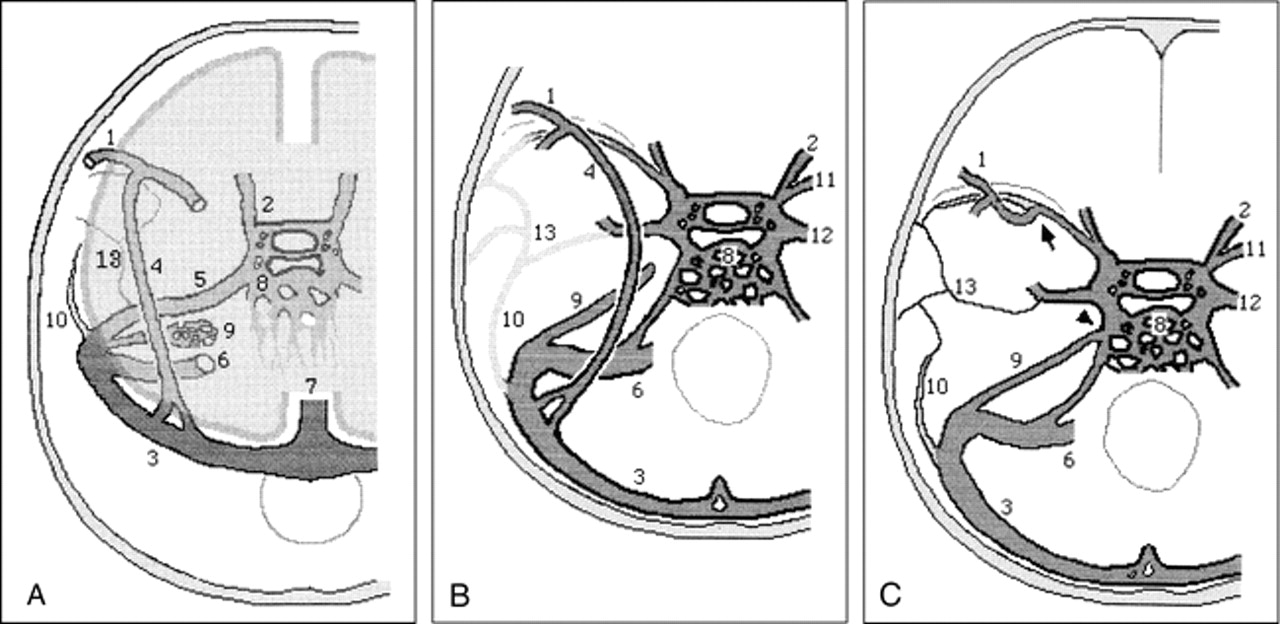This scientific diagram depicts the brain and its associated blood vessels in a detailed, black and white illustration. The image is divided into three sections labeled A, B, and C, from left to right, with each section progressively zooming in on particular aspects of the brain's vascular system. Section A shows a broad view of the brain's structure, while section B provides a closer look at the central area, and section C focuses on the intricate vessels underneath that central section. 

The diagram's hard black border is shaped partially to resemble a skull, further contextualizing the anatomical components presented. Each section's elements, including the tubes and pathways, are colored in dark and light grays. Numbers are used to mark specific areas within each section, ranging from 1 to 18, although no legend is provided to explain these numerical designations. The overall illustration attempts a 3D style to enhance the depiction of the complex vessel network within the brain.